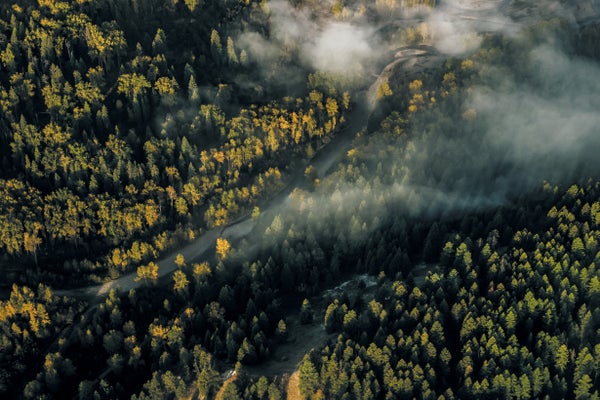This aerial photo captures a densely wooded forest, with a winding river running through it, starting near the bottom left corner and meandering toward the upper right. The forest landscape is notably hilly, with a steep drop or cliff featured on the right-hand side. The trees, though varied, primarily consist of a mix of evergreens and some deciduous trees whose yellowish leaves hint at the season. The early morning sunlight is beginning to illuminate the tree tops, casting a golden hue, while much of the forest remains cloaked in shadow. A delicate layer of morning mist or fog drifts across the scene, particularly where the sun’s rays are breaking through, adding an ethereal quality. Sparse areas suggest past disturbances or tree removal, and low, wispy clouds hover above the river. Although the lighting and shadows make some details indistinct, the overall picture reveals a breathtakingly serene landscape caught at the break of dawn.